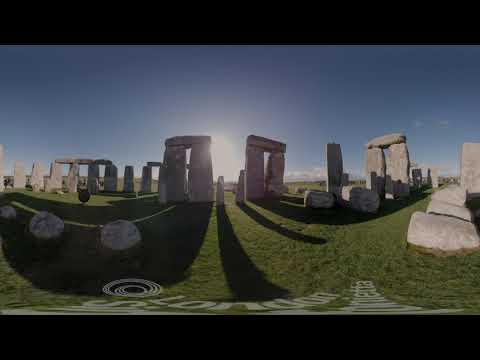This image captures a wide-angle, distorted view of Stonehenge taken with a fisheye lens, giving the ancient stone structures an exaggerated curvature. The foreground features a grassy field, typical of the site’s setting, while the background showcases a clear, sunny sky. Stonehenge's iconic vertical columns, topped with horizontal stones forming arch-like shapes, dominate the center of the photo, casting their famous shadows. Despite some stones lying on the ground, the primary structure resembles the mathematical pi symbol. The lower edge of the image contains a distorted watermark reading "L-O-N-D-O-N." There is a black border framing the entire scene. The colors visible in the image include black, blue, white, gray, tan, brown, and green, adding to the picturesque and timeless quality of this outdoor, midday snapshot.